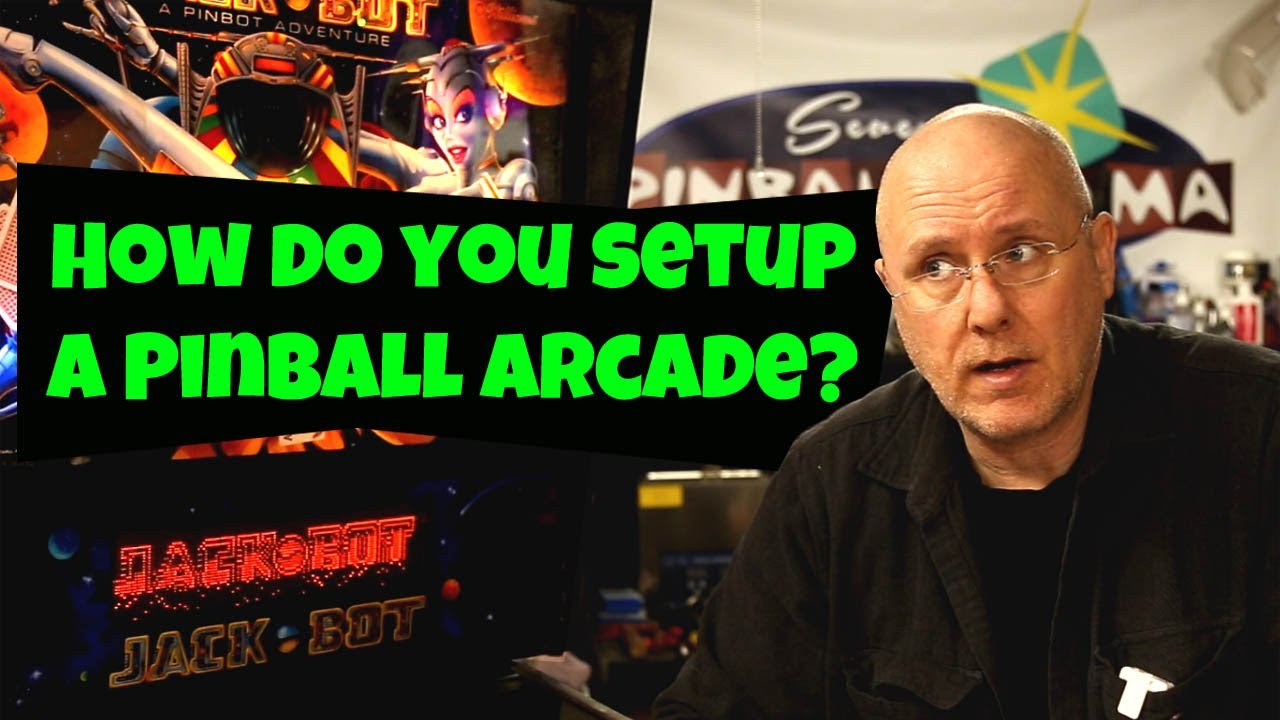The image is a detailed, rectangular photograph taken indoors, measuring approximately six inches wide and three inches high. It captures a middle-aged Caucasian man, who is likely in an arcade setting. The man, who has a bald head with sparse white hair near the temples and light wire-framed glasses, is visible from the chest up. His expression, highlighted by slightly raised eyebrows and a wrinkled forehead, shows him with a mouth slightly open, as if in mid-conversation or thought. He has a bit of a five o'clock shadow and mustache. He is dressed in a black t-shirt layered under a black, open, long-sleeve button-up shirt.

Dominating the center of the image, in bold green letters, the text "How do you set up a pinball arcade?" stands out, suggesting an instructional theme. To the left of the man and partially behind this text, is an arcade machine labeled "Jackbot," themed possibly around sci-fi elements with colorful characters and references to "jackpot." The background also includes other pinball machines or video games, along with a noticeable sign on a white wall that seems to read "SCV pinballorama," reinforcing the arcade environment.

Overall, the scene suggests the man might be involved in the pinball arcade business, possibly discussing or providing insights on setting up an arcade, in what could be an instructional or interview setting.